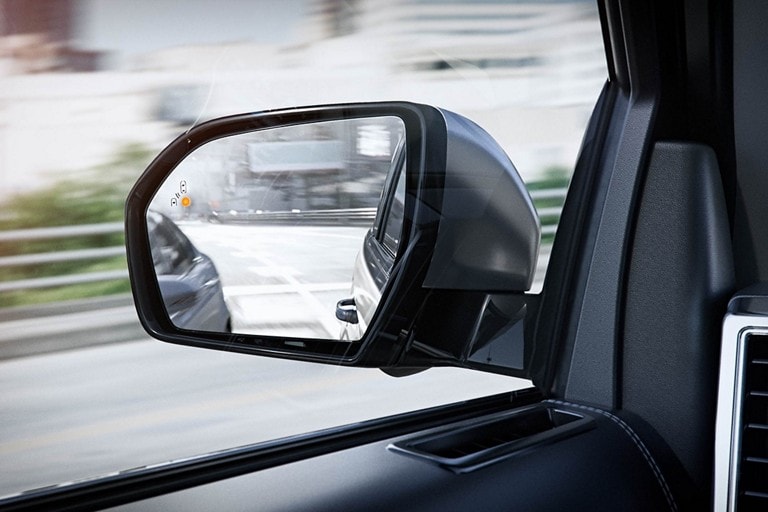This image is taken from inside a moving vehicle, specifically from the driver's side. The focal point is the side rear view mirror, positioned towards the left of the image, and the rest of the car's interior, which is sleek with a black finish, occupies the bottom left to the bottom right corner. The mirror reveals a small, grey car in its reflection. The background seen through the mirror is blurry, indicating motion, and features some greenery and white buildings, along with horizontal bars of a rail near the road's end. The overall scene outside the window also appears blurred, emphasizing the car’s movement. The color palette includes a metallic gray, black, dark gray, matted black, orange, and green. Additionally, a vent can be seen on the lower right side of the door inside the car.